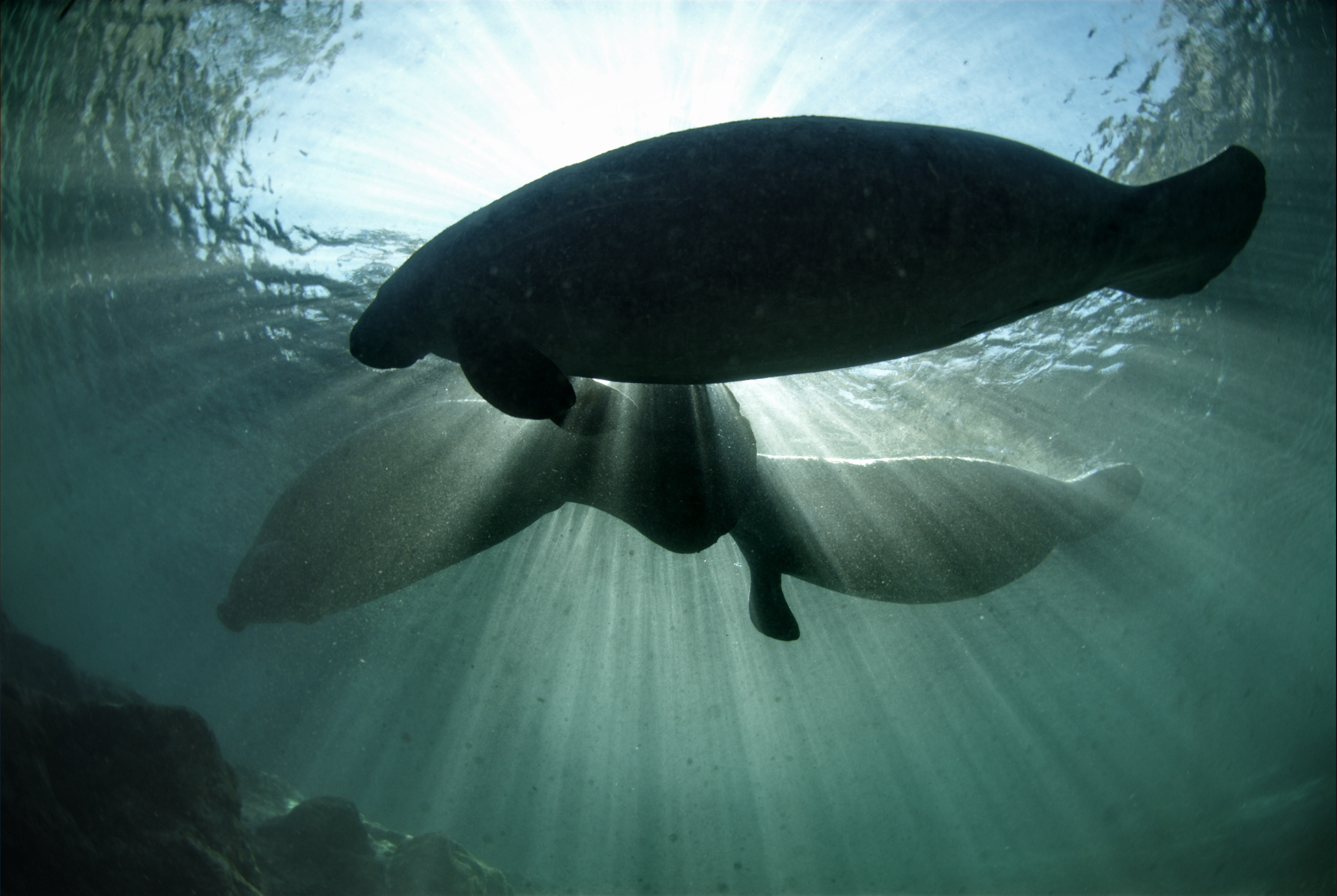Captured by a skilled wildlife photographer, this enchanting underwater image showcases a serene, sunlit scene in the ocean or sea. The blue and green hues of the water are illuminated by sunlight filtering through the surface, casting a beautiful, even dispersion of light rays that penetrate deep into the aquatic environment. At the bottom, scattered rocks and blurred plant life add texture to the scene. Dominating the image, two large marine creatures—resembling black and green colored whales—swim gracefully, their figures casting shadows on the ocean floor. Accompanying them, a group of turtles can be seen gliding effortlessly through the water, enhancing the scene's vibrant, underwater ecosystem.